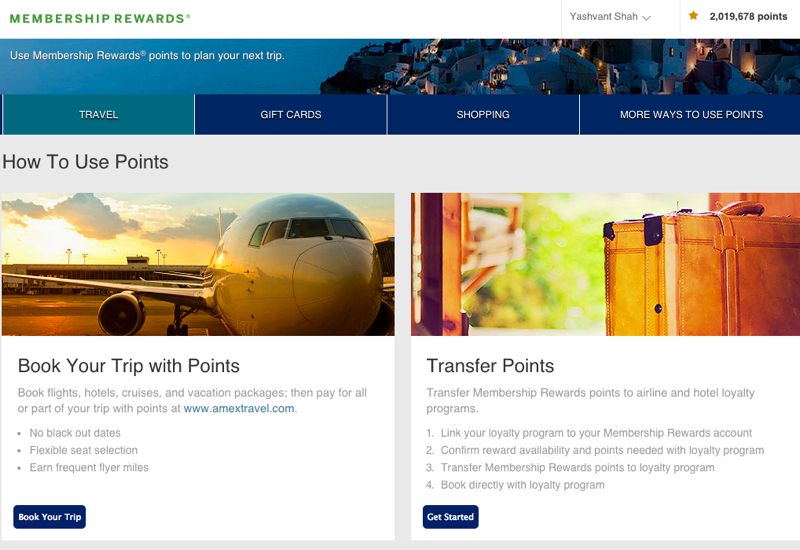The image is a screenshot of a webpage dedicated to membership rewards. The top of the page features a green header with the text "Membership Rewards." The background of the page is white. On the right side, there is a dropdown menu associated with the name "Yashvant Shaw," indicating that the user has accumulated 2,019,678 points, highlighted by a star icon.

Below this section, a prominent blue banner with white text encourages users to "Use Membership Rewards Points to Plan Your Next Trip." Below this main banner are several tabs for various options to use points: "Travel" on a lighter blue tab, followed by "Gift Cards," "Shopping," and "More Ways to Use Points" on darker blue tabs.

Further down, a white banner titled "How to Use Points" features images and calls to action. One image depicts an airplane at an airport during a sunset, with clouds in the background and text reading "Book Your Trip with Points," where "Book Your Trip" is in blue. Another graphic shows a suitcase positioned in a doorway, accompanied by the message "Transfer Points" and a blue "Get Started" button.